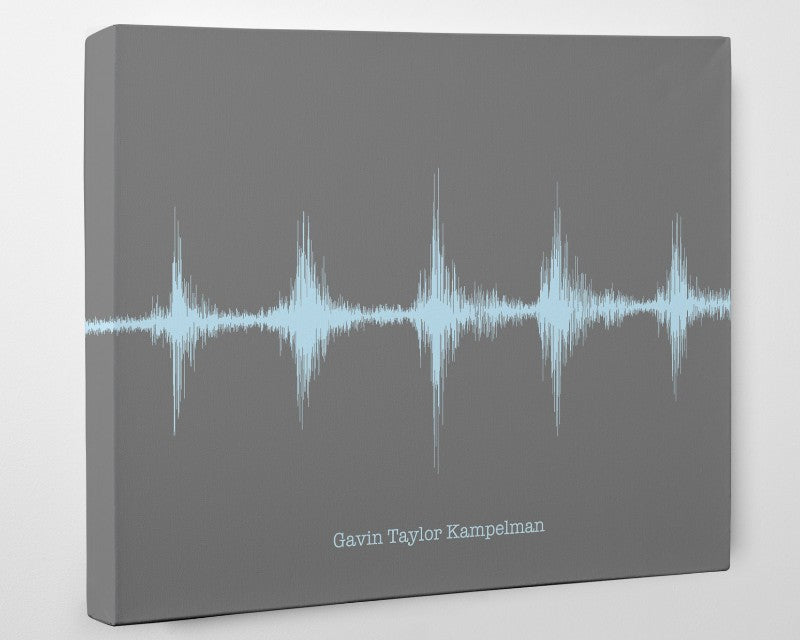This image showcases a dark gray canvas artwork featuring a light baby blue sound wave design. The wave begins in the middle of the left side, wraps around the corner, and extends through the center of the canvas to the right edge. The sound wave pattern consists of sharp peaks and smaller spikes, resembling an audio signal or electrocardiogram pulses. At the bottom of the canvas, the artist's name, "Gavin Taylor Campbellman," is prominently displayed in the same light blue color as the wave, clearly written: Gavin with a G.